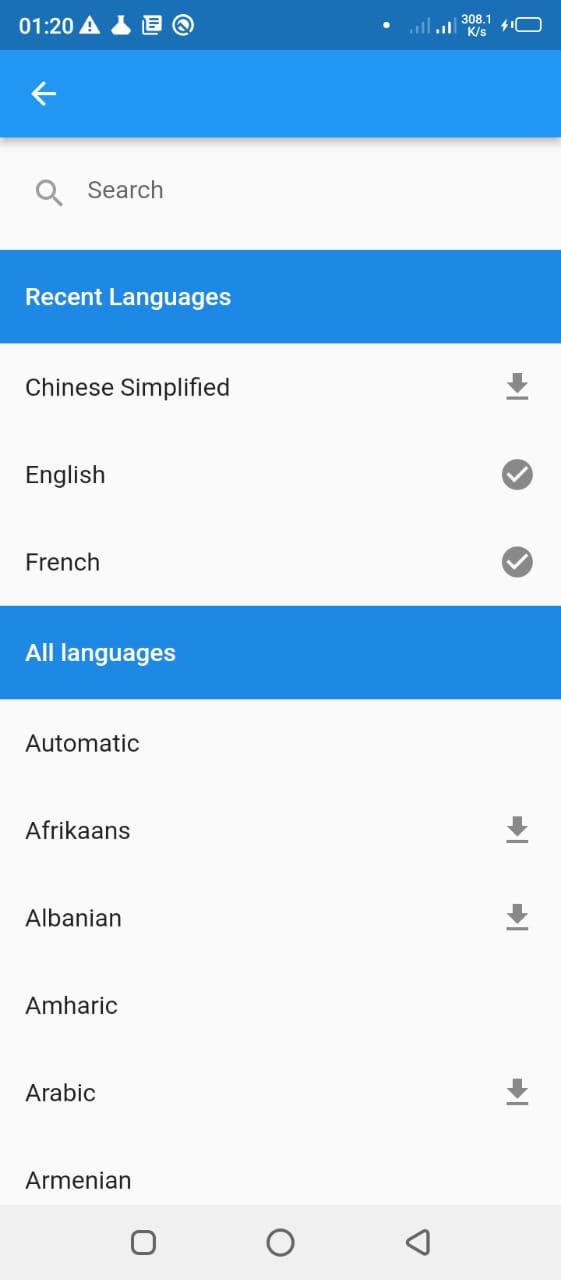The screenshot appears to be from a tablet or smartphone device, showcasing a language settings page within an application. The status bar at the top indicates the time "1:20" alongside a caution sign, an almost depleted battery icon with a charging symbol beside it, and visible signal strength indicators. Thematically, the interface predominantly features shades of blue, light gray, and white, with both black and white text for contrast.

At the very top, there is a blue banner containing a white back button. Below this banner, there is a search bar adorned with a magnifying glass icon and the placeholder text "Search." Following the search bar, a blue section labeled "Recent Languages" displays options in white text: Chinese (Simplified), English, and French.

The next section titled "All Languages" lists various languages such as Automatic, Afrikaans, Albanian, Amharic, Arabic, and Armenian. Each language option has a downward-pointing arrow next to it, likely indicating a dropdown menu or download option, and some languages have a checkmark, suggesting they are already selected or downloaded.

At the bottom of the screen, the three standard navigation icons of an Android device are visible, including the back, home, and recent apps buttons. This detailed layout confirms that the screenshot is from a language settings menu within a mobile application, providing users with a variety of language options to choose from.